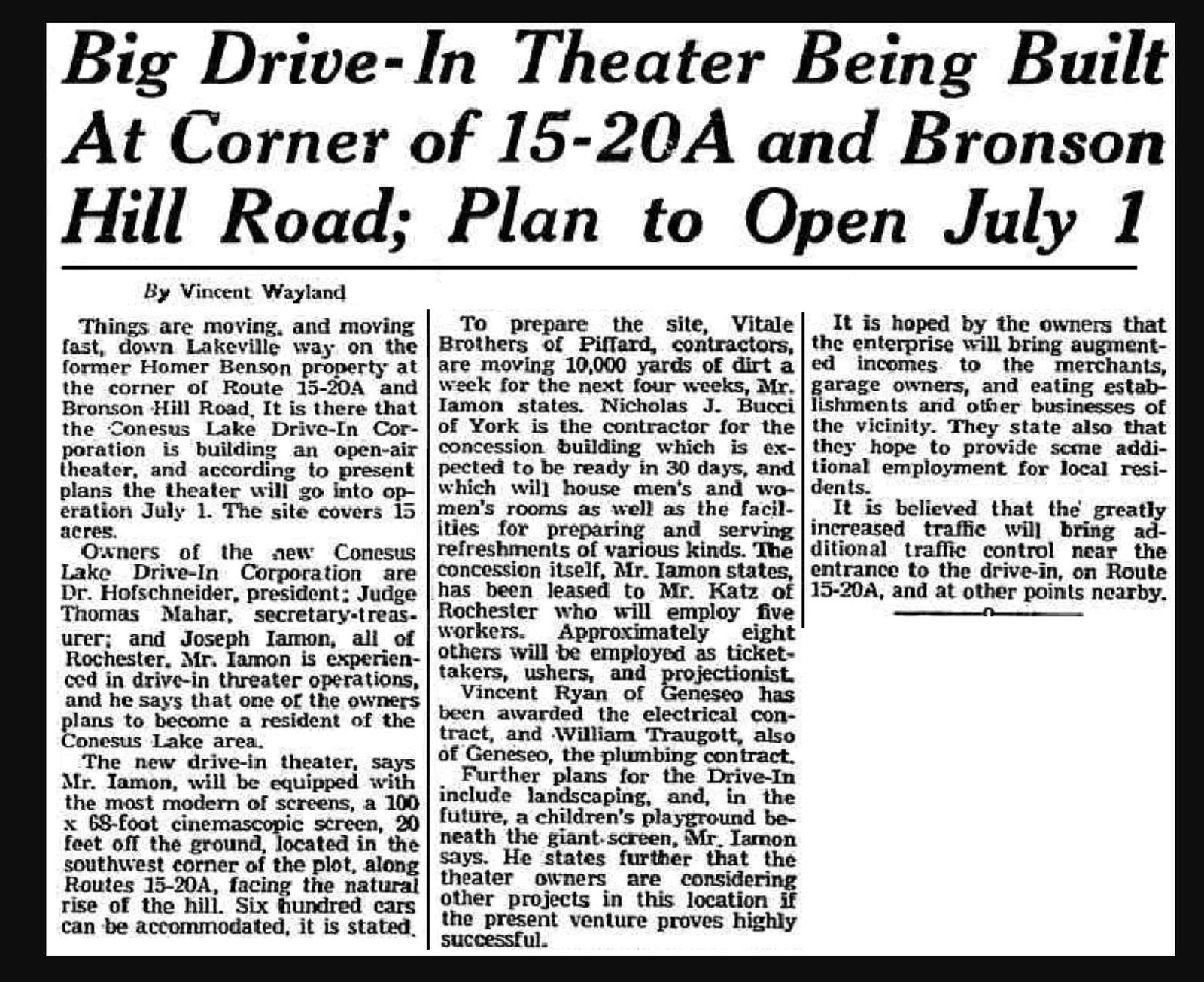The image is a black and white news clipping from a newspaper, outlined with a black border and filled with very small print. The title reads, "Big Drive-In Theater Being Built at the Corner of 15-20A and Bronson Hill Road, Planned to Open July 1st." The article, written by Vincent Whelan, details the development of a new open-air theater by the Consensus Lake Drive-In Corporation on the former Homer Benson property at the intersection of Route 15-20A and Bronson Hill Road. Things are progressing quickly at the 15-acre site, with traffic expected to increase significantly, requiring additional traffic control near the entrance. The owners of the Consensus Lake Drive-In Corporation are Dr. Hemsfield (President), Judge Thomas Madder (Secretary-Treasurer), and Joseph Weyland, all of Rochester. Mr. Weyland, experienced in drive-in theater operations, mentioned that one of the owners plans to become a resident of the Consensus Lake area. The entire article spans 7-8 paragraphs, focusing on the anticipated economic boost for local merchants, garage owners, and eating establishments, as this much-awaited drive-in theater aims to open on July 1st.